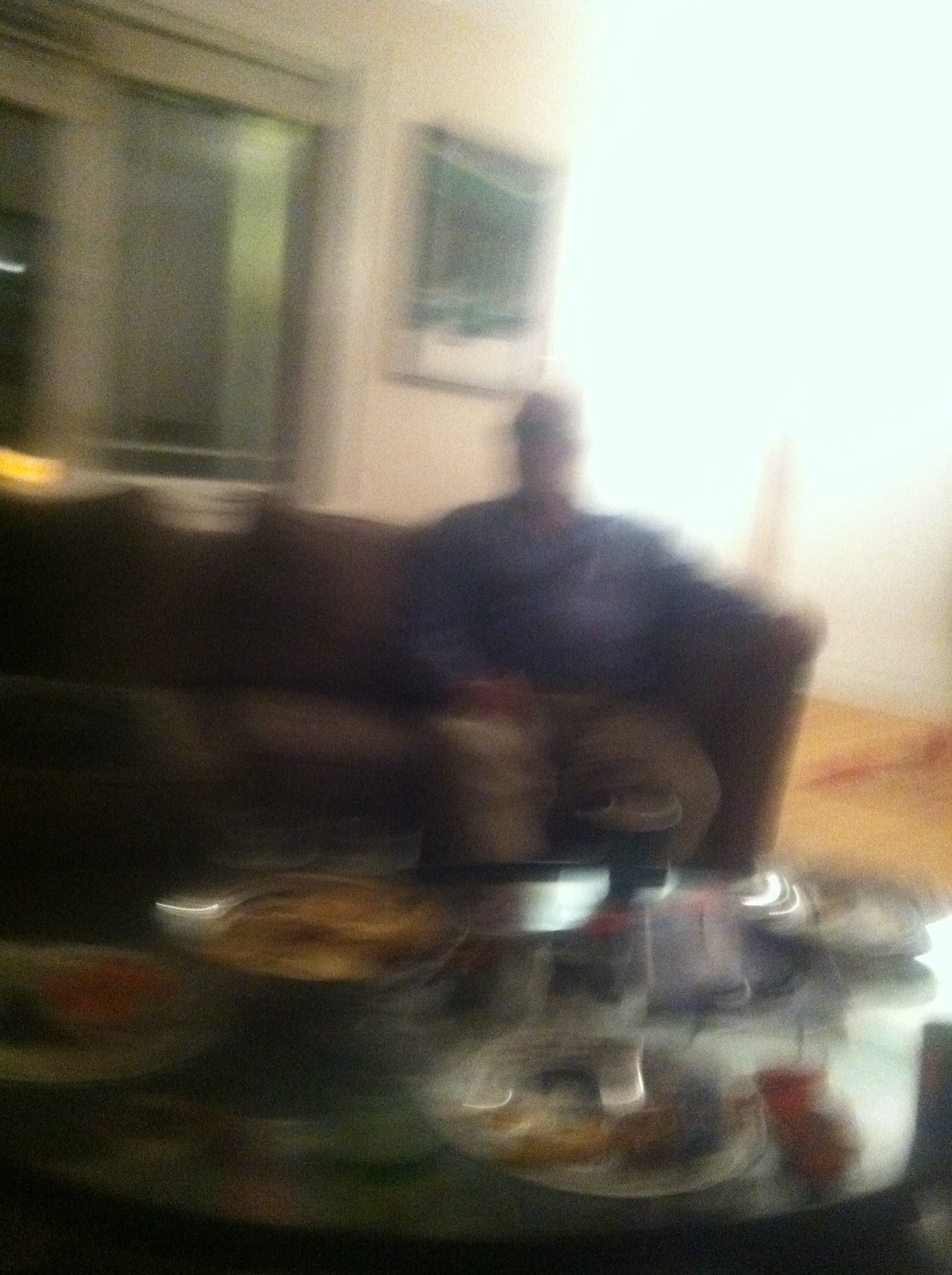In this blurry, washed-out photograph, we get a glimpse of a cozy sitting room where a middle-aged man with dark brown skin is seated. He is comfortably positioned on the far left of a dark brown fabric couch, wearing a blue long-sleeve shirt and khaki pants, possibly with a hat on. His left arm rests on the couch's armrest, while his right hand is placed on his knee. A glass coffee table in front of him is cluttered with various indistinct platters and bowls of food, some of them suggesting a celebration, perhaps a birthday or dinner gathering. The background reveals a window with white trim and a painting in tones of green, white, and blue on the upper left wall. A bright, diffuse light dominates the right side of the image, obscuring the details with a sky-blue blur, likely due to an open doorway or another window. The floor beneath is brown, contributing to the warm ambiance of the room.